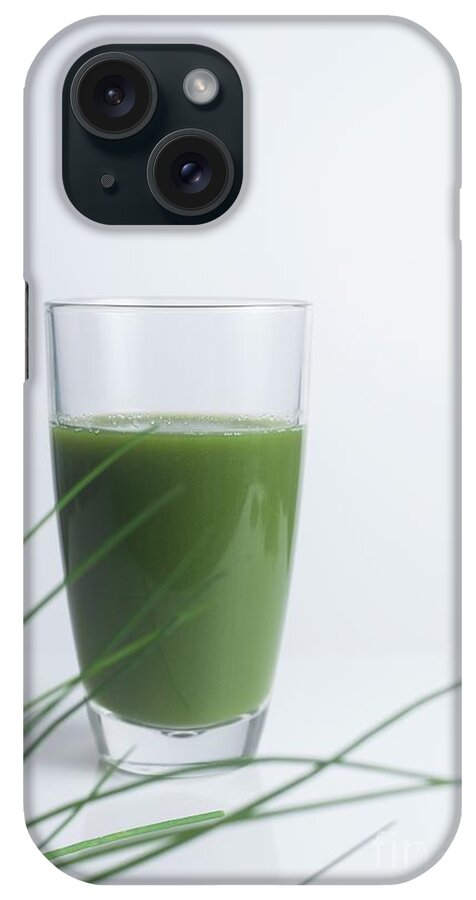The image depicts the back of a cell phone, likely an iPhone, encased in a phone cover. The phone case is primarily white or off-white with a clean, minimalistic design. In the upper left-hand corner of the case, there's a distinctive black square with rounded edges housing dual camera lenses and a flash. Below this, a clear glass filled with a vibrant green juice takes central focus. Surrounding the glass, blades of green grass extend outwards, enhancing the natural theme. The entire setup is on a plain white background, making the details of the phone case and its design elements stand out clearly. The phone case itself features smooth, rounded corners and is visually striking with its realistic photographic print and light gray shadow effects.